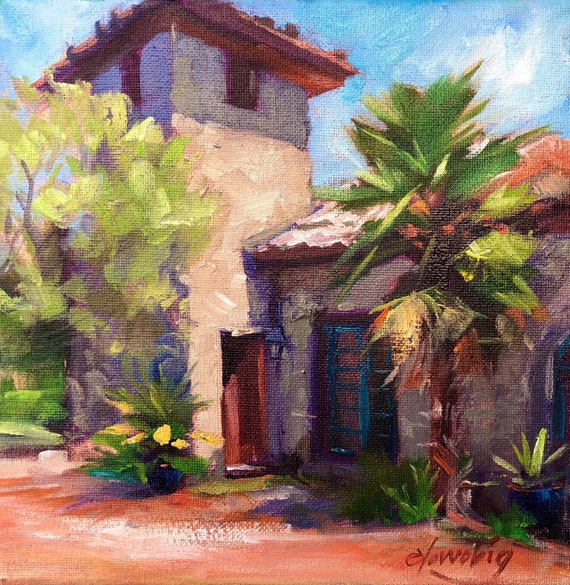This vibrant, simplistic oil painting captures a charming Mediterranean-Caribbean style cottage. The cottage features adobo or clay walls in a pinkish stucco finish, capped with red clay tile roofs. Despite its lack of intricate details, the painting is rich in texture and color, likely done in acrylic or oil. In front of the cottage stands a prominent palm tree along with other tropical plants and greenery. A dirt walkway leads up to the blue-windowed, multi-pane brown door, adding to the rustic appeal of the scene. Surrounding the house, bursts of blues, greens, and yellows blend harmoniously with the sandy clay tones of the cottage walls. In the lower right-hand corner, the artist has signed the piece, though the exact name is difficult to decipher. The painting, while not realistic, beautifully conveys the essence and shapes of its idyllic setting.